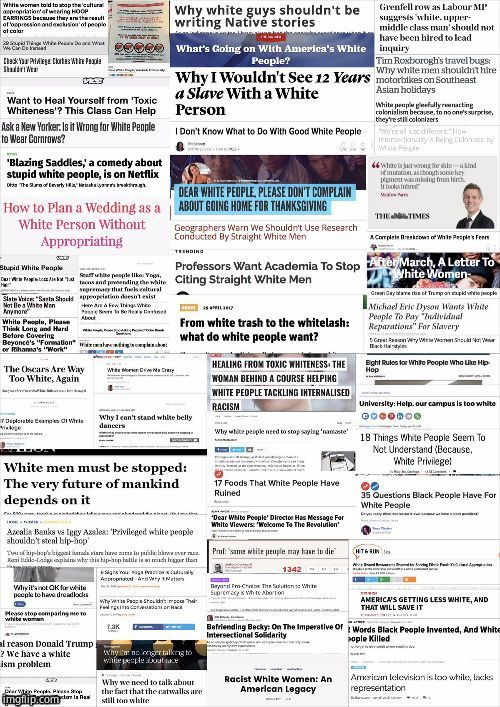This image features a digital collage resembling old newspaper ads, organized in three uneven columns filled with article titles. The titles are clearly readable in some parts, while others are blurred, suggesting a focus on themes related to race and cultural appropriation. Here are several titles that stand out:

- **Want to Heal Yourself from Toxic Whiteness? This Class Can Help**
- **Is It Wrong for White People to Wear Cornrows?**
- **Blazing Saddles: A Comedy About Stupid White People is on Netflix**
- **How to Plan the Weather as a White Person Without Appropriating**
- **Stupid White People: The Oscars are Way Too White Again**
- **Why Can’t I Stand White Belly Dancers?**
- **White Men Must Be Stopped: The Very Future of Mankind Depends on It**
- **Azalea Banks Versus Iggy Azalea: White Privilege in Hip-Hop**
- **White People Shouldn't Steal Hip-Hop**
- **Why We Need to Talk About the Fact That Cat Walks Are Still Too White**
- **Racist White Women: An American Legacy**
- **Befriending Becky: Imperatives of Intersectional Solidarity**
- **Dear White People Director Has a Message for White Viewers: Welcome to the Revolution**
- **17 Fools that White People Have Been Ruined By**
- **35 Questions Black People Have for White People**
- **America's Getting Less White and That Will Save It**

Presented in differently colored texts, the collage brings a striking and provocative commentary on white culture and racial issues in contemporary society.